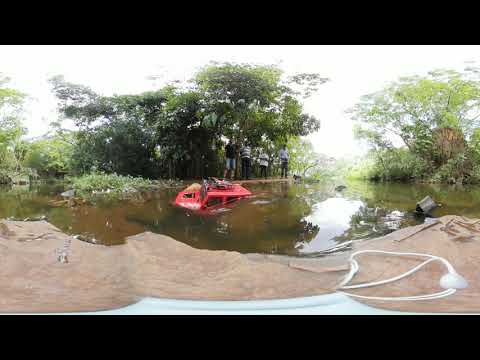The photograph depicts an outdoor scene during the daytime, characterized by a somewhat swampy and marshy environment with a body of water that appears more like a flooded embankment or ravine. Dominating the center of the image is a nearly submerged red SUV, its roof and hood barely visible above the murky, brown water. The water seems relatively clear, revealing rocks at its bottom despite its color.

In the background, on a dry patch of land across the water from the camera, stand four men, presumably with dark skin. Their precise features are difficult to discern, but they are dressed casually, some even in shorts, suggesting a warm climate. These men appear to be observing the partially submerged vehicle with interest, possibly indicating that the SUV encountered trouble due to unexpectedly deep water, leading to its current predicament.

In the foreground, closer to the viewer, the land consists of dry dirt, suggesting the opposite embankment remains unaffected by the flood. The environment around them includes trees and a cloudy, white sky, providing a sense of a natural, yet disrupted landscape.